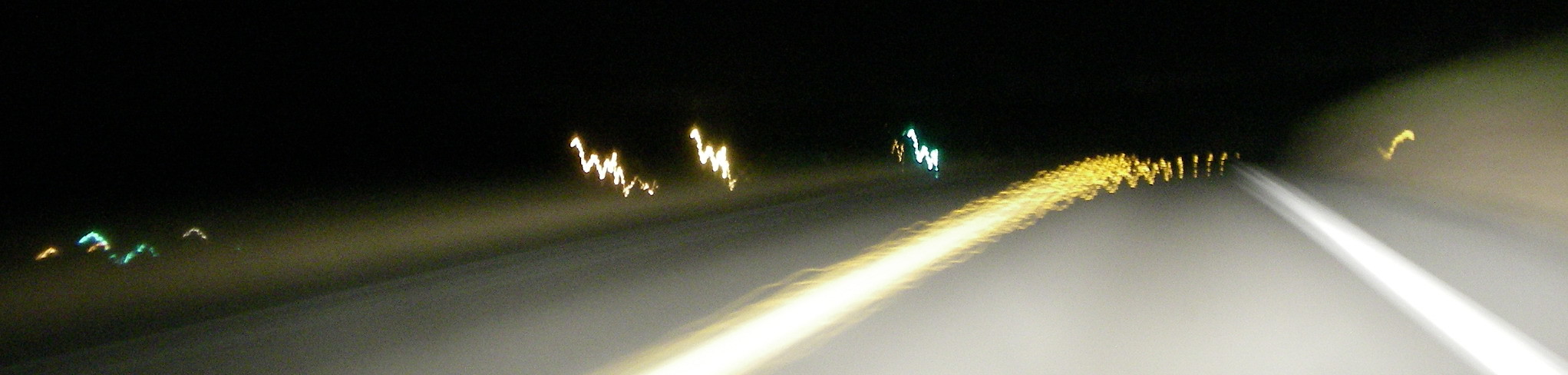This nighttime panoramic photograph captures an intriguing scene that combines both surreal light effects and a sense of depth. The focal point is a road with a distinct yellow line running centrally, appearing almost luminous as it stretches off into the distance. On either side of the road, white lines demarcate the path, with the left one featuring squiggly, lightning-like light patterns. The right side of the image seems to transition into what might be a wall or hill, contributing to an impression that the scene could be inside a tunnel. The photo's special lighting effects and blurriness add to its surreal quality, with scattered squiggly lines of light—some blue, some white—providing additional points of visual interest against the otherwise dark background. The scene is both mesmerizing and disorienting, using a combination of unique lens effects and lighting to transform a simple road into a dynamic visual spectacle.